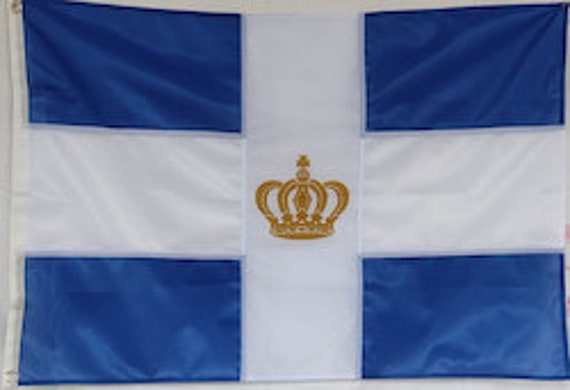This image is a color photograph of a flag with a distinctive design. The flag has a blue background featuring a large white cross that intersects in the center, creating a prominent plus sign. At the intersection of the white stripes, there is a detailed illustration of a gold crown. The upper left corner of the flag has a metal grommet, indicating it can be attached to a pole. The material of the flag appears to be shiny, resembling polyester. The flag is not affixed to anything in the picture and seems to be hanging on a wall. Despite initial confusion about its origin, it was clarified that this is a unique or possibly stylized version loosely inspired by the Greek flag, rather than being Scandinavian. The overall scene conveys a sense of a well-crafted, possibly ceremonial flag.